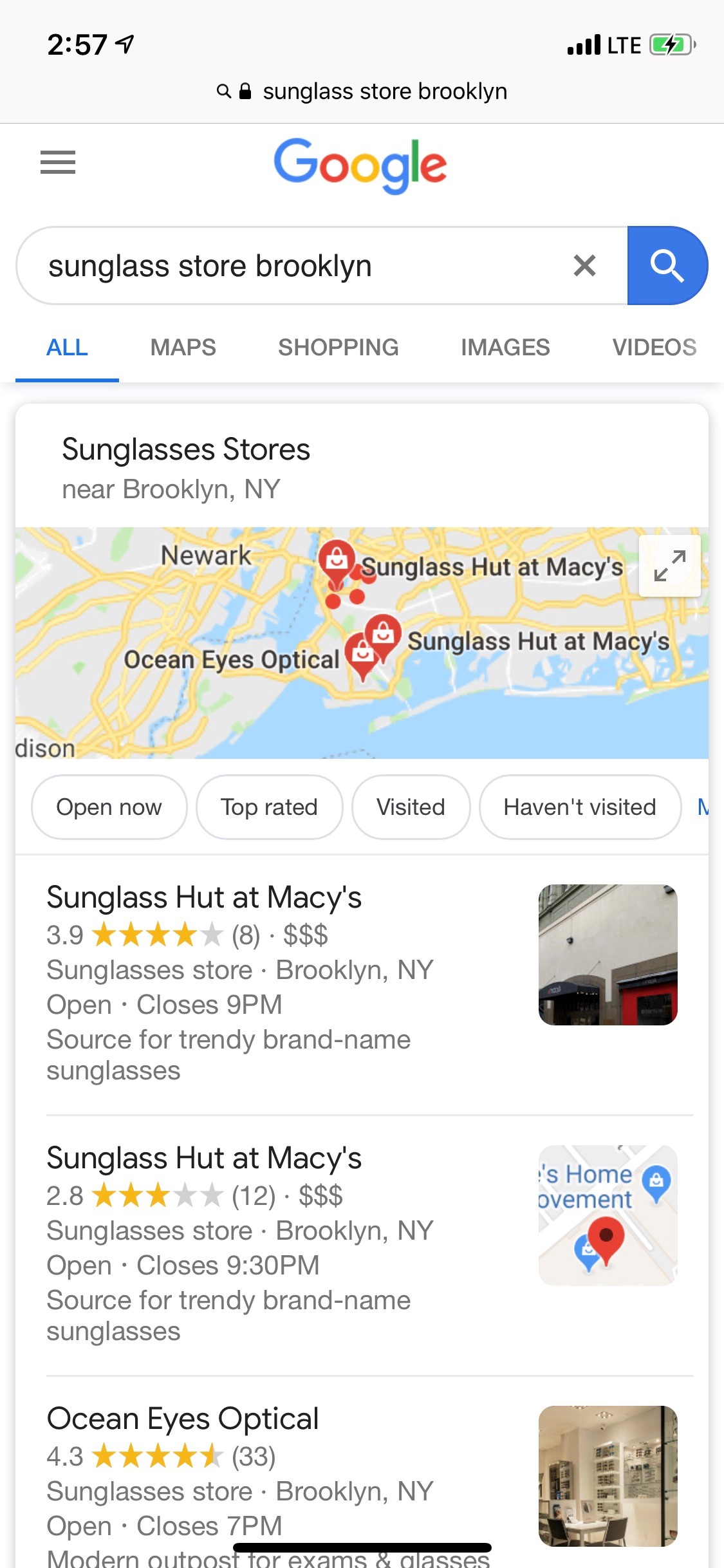A detailed caption for the provided image:

"This is a screenshot taken from a Google search on a smartphone. The top of the screen displays the status bar showing a time of 2:57, a battery icon, and connection status indicating LTE coverage. Below, a search bar with the query 'Sunglass Store Brooklyn' is visible, followed by the Google logo in its signature blue, red, yellow, blue, green, and red colors.

Directly underneath, another search bar mirrors the same query 'Sunglass Store Brooklyn', with tab options including 'All' (which is currently selected), 'Maps', 'Shopping', 'Images', and 'Videos'. The search results include a map of Brooklyn with various sunglasses store locations marked.

Highlighted search results show:
1. **Sunglass Hut at Macy's**:
   - Rating: 3.9 out of 5 stars
   - Reviews: 8
   - Price: $$$
   - Location: Brooklyn, New York
   - Status: Open, closes at 9 PM
   - Description: Source for trendy brand name sunglasses

2. **Sunglass Hut at Macy's** (another listing):
   - Rating: 2.8 out of 5 stars
   - Reviews: 12
   - Price: $$$
   - Location: Brooklyn, New York
   - Status: Open, closes at 9:30 PM
   - Description: Source for trendy brand name sunglasses

3. **Ocean Eyes Optical**:
   - Rating: 4.3 out of 5 stars
   - Reviews: 33
   - Location: Brooklyn, New York
   - Status: Open, closes at 7 PM
   - Description: Modern outpost for eye exams and glasses

The search also includes filter tags reading 'Open now', 'Top rated', 'Visited', and 'Haven't visited'.